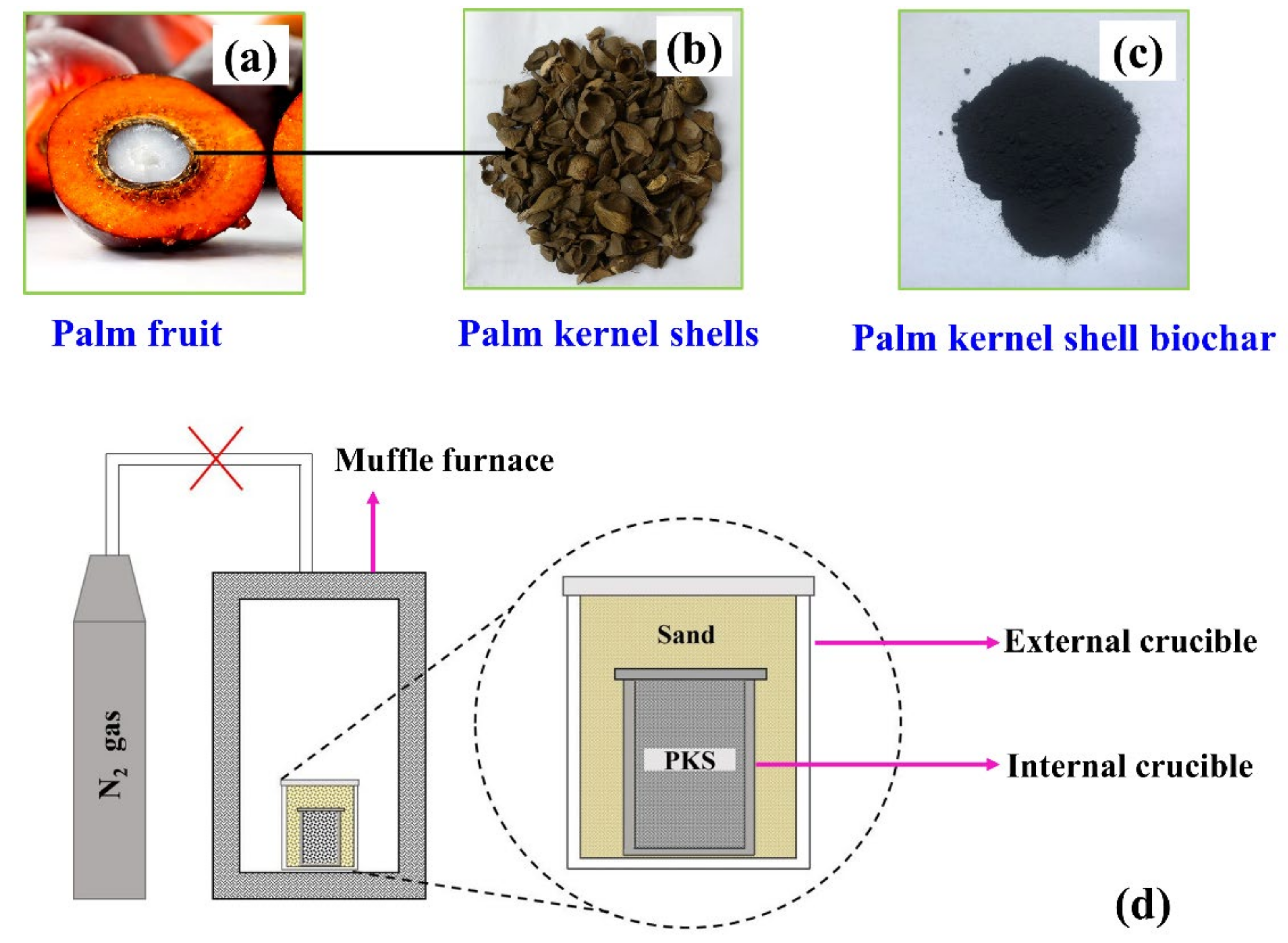This image serves as an informational chart detailing the process of transforming a palm fruit into palm kernel shell biochar using a muffle furnace. At the top, it features three interconnected stages labeled A, B, and C. The first image (A) displays a cut-open palm fruit, revealing its colorful insides with an orange, red, and yellow exterior and a white center. Connecting to this, the second image (B) shows the extracted palm kernel shells, resembling dark brown, greenish wood shavings. The third image (C) presents the final product: black, dusty palm kernel shell biochar.

The lower section of the chart shifts focus to a technical sketch of a muffle furnace setup, labeled D. The sketch details a system where nitrogen gas (N2) from a silo is funneled into the furnace. This muffle furnace is illustrated with an expanded view showing its construction and operation. It is surrounded by sand and features an external crucible that forms the outer wall, and an internal crucible located at the furnace's core. This diagram provides a comprehensive understanding of how the palm kernel shells are processed into biochar within the furnace setup.